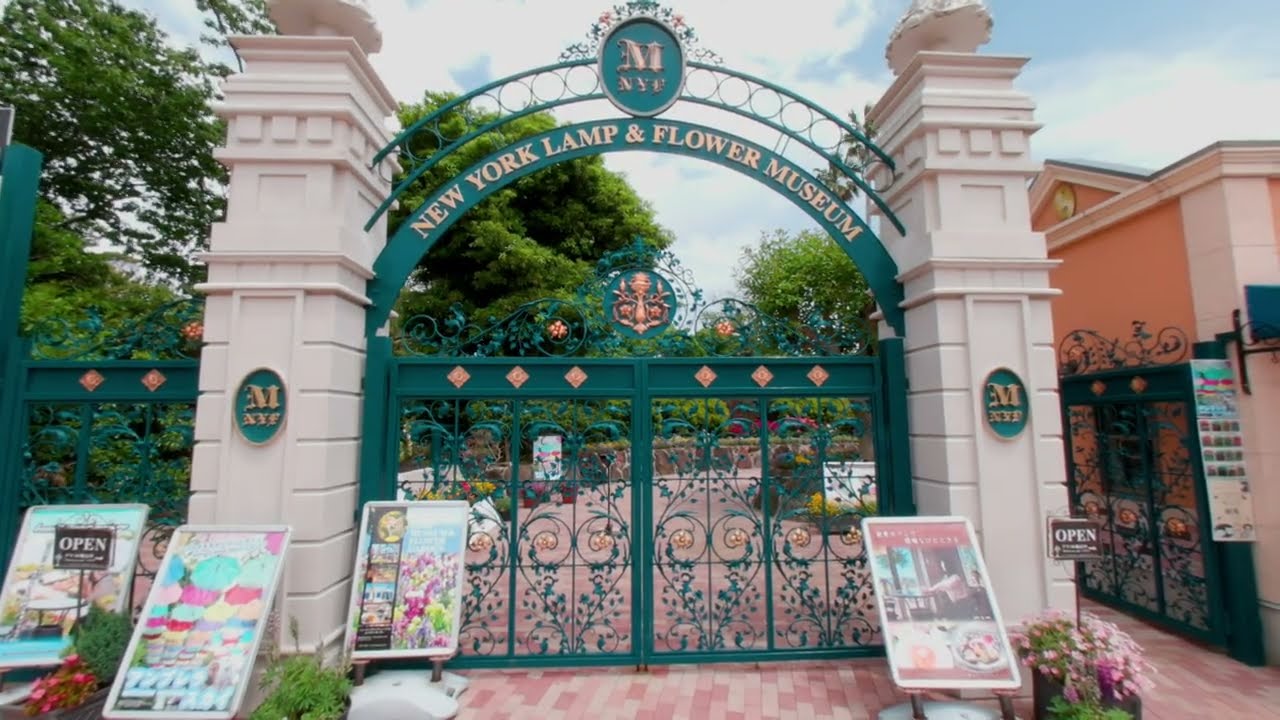This image showcases the ornate entrance gate of the New York Lamp and Flower Museum. The gate is made of green scrolled ironwork, adorned with elegant gold and pink lettering that spell out "New York Lamp and Flower Museum" in an arched pattern, complemented by an emblem featuring the letters "MNYF". The entrance is flanked by two tall, off-white concrete pillars crowned with mushroom cap designs. Beneath a sky that's a mix of white and blue with many clouds, the scene is captured during the daytime.

The pathway leading from the gate is a beautifully paved light red and pink cobblestone path, smooth and turning to the right, guiding visitors toward the museum. To the left of the path inside the gate, lush, flourishing trees provide a natural canopy. Multiple signs and posters are displayed along the entrance, likely detailing exhibits or museum attractions, with a small black and white sign indicating that the museum is open. The right column also features a smaller gate, perhaps for a guest entrance. The overall setting exudes a welcoming and picturesque ambiance.